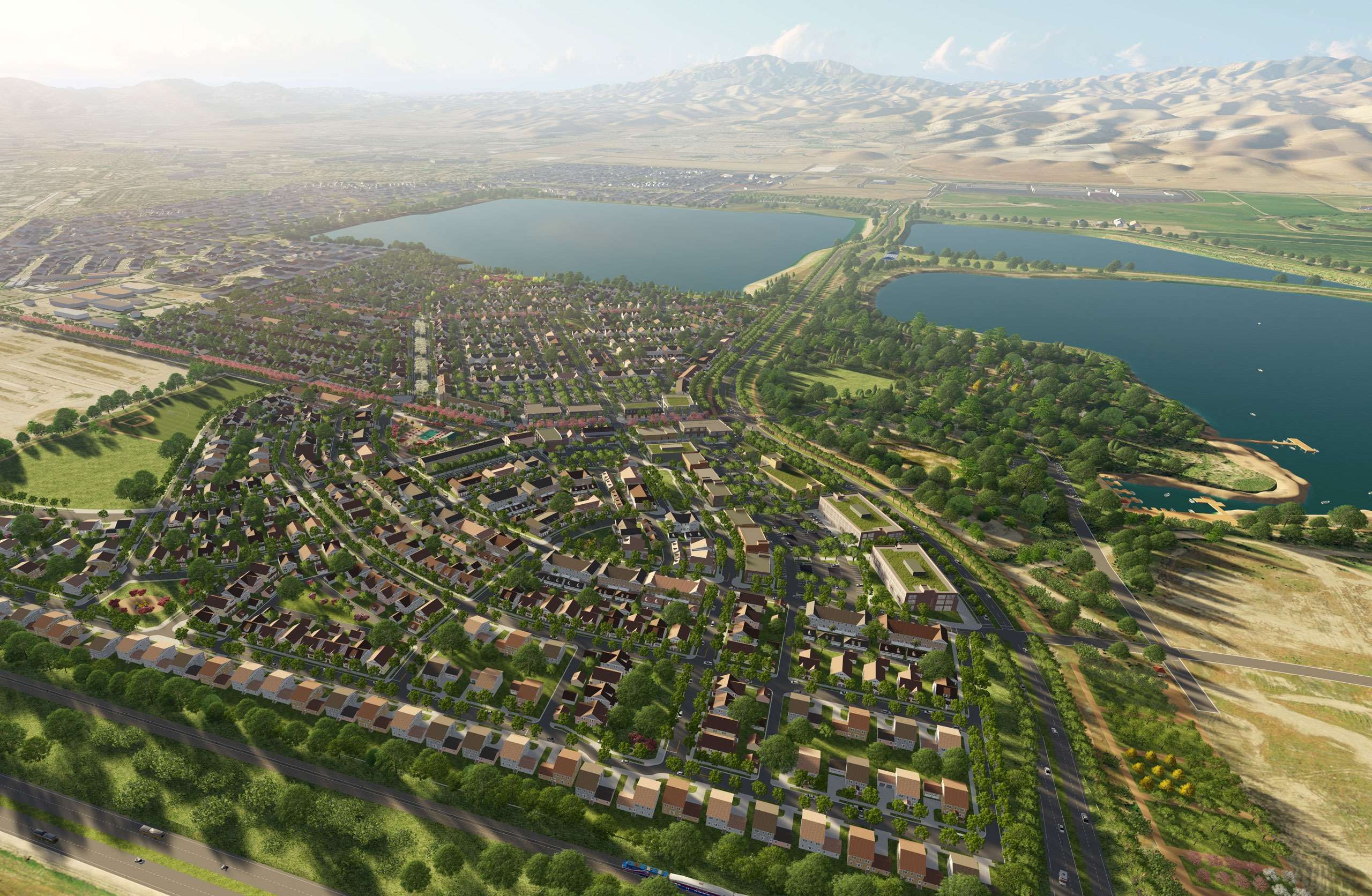The image is an aerial view of a small city or suburban town intertwined with nature. The landscape showcases lush green vegetation and multiple water bodies, including a square-shaped and a triangular-shaped body of water separated by a thin piece of land. Roads crisscross the town, connecting various structures—ranging from single-family homes with tan, brown, or black roofs to larger apartment or commercial buildings. In the foreground, a subdivision of houses is visible, with one area featuring what appears to be a swimming pool, possibly part of a recreational center. Docks line the right side near the water, highlighting the town's proximity to the bay. The background reveals an elevated mountain ridge under clouds with sun rays filtering through, giving way to a more arid, less developed landscape. The entire setting, though urban with its organized roads and buildings, blends seamlessly with natural elements, presenting a picturesque view as if captured from a bird's eye perspective.